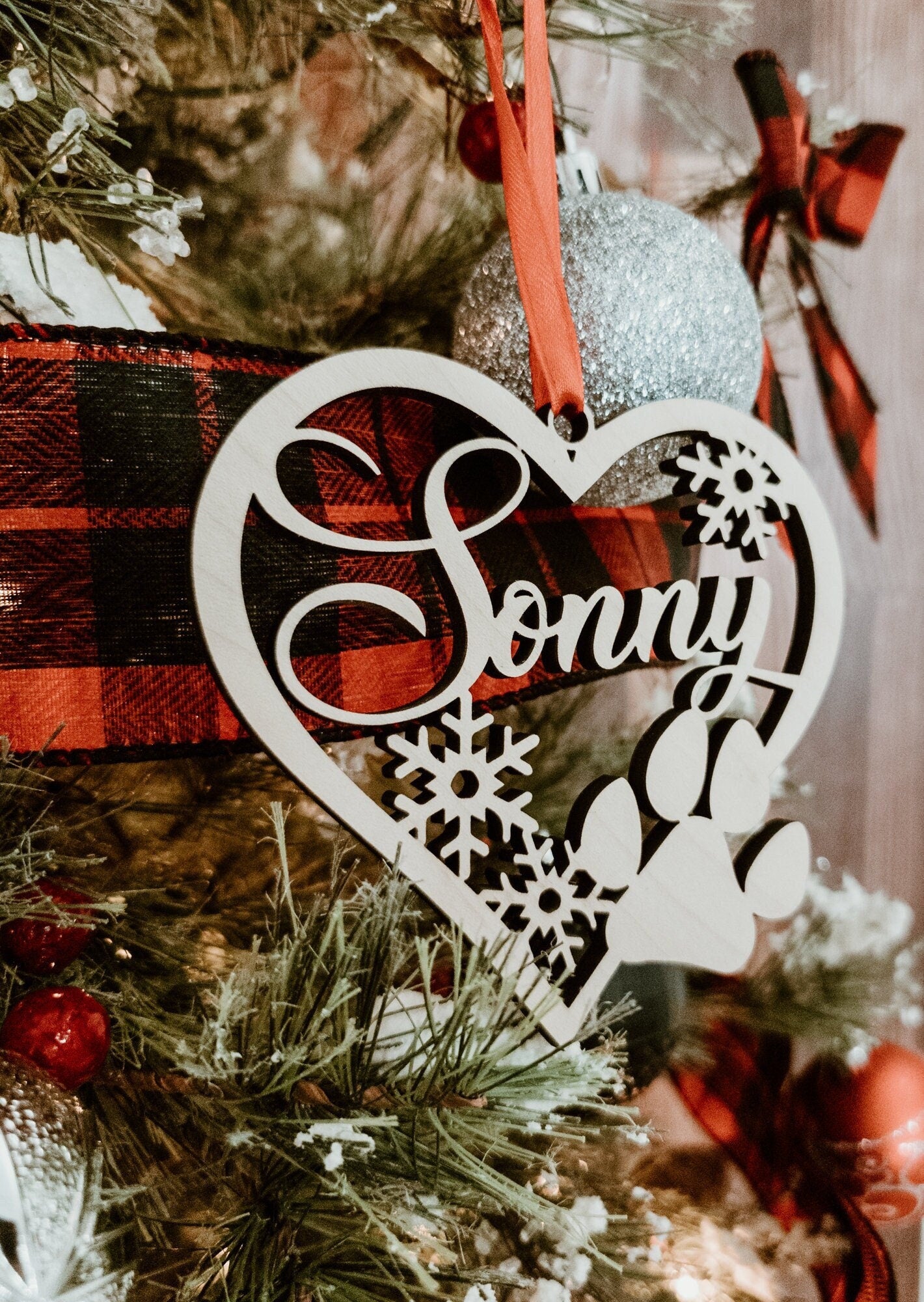In this vertical, rectangular image of a Christmas display, a heart-shaped ornament prominently hangs in the foreground. The heart, crafted from metal and adorned with the word "Sunny," is a tribute to the family's dog. Detailed markings on the heart include two snowflakes positioned at the top right and bottom tip, and a central large paw print. It dangles from a red ribbon in front of a red and black plaid blanket draped across the middle of the scene. Surrounding the heart are greenery and long evergreen needles, indicating it is part of a Christmas tree adorned with festive decorations. A spherical red ornament with silver accents is visible at the bottom right, further enhancing the holiday decor. Realistic snow adds a touch of wintry charm to this heartwarming setup.